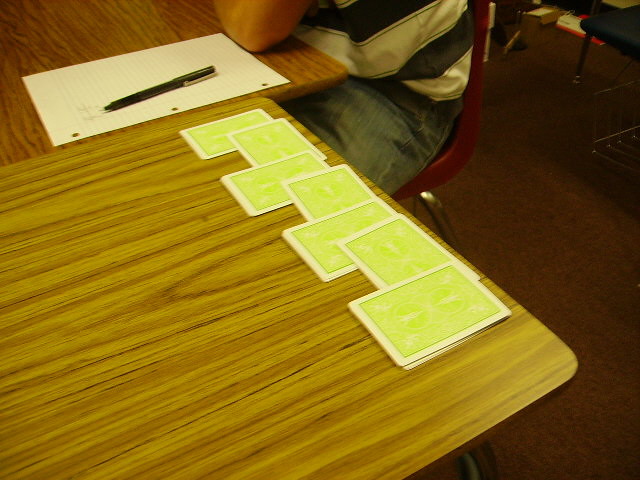In this photograph, we see a pair of tables joined together, reminiscent of those found in schools or public libraries. The tables feature curved, tapered metal legs. Adjacent to the tables is a red plastic chair, also supported by shiny metal legs, placed on a brown carpeted floor. The shot captures the corner of one table in the foreground and a portion of the adjacent table behind it. On the table at the back rests a sheet of notebook paper with a pen lying on top. A person is seated in the red chair, wearing blue jeans and a white and blue striped shirt. Their elbow is propped on the table as they intently gaze down at the paper, appearing as though they might have been doodling or writing.

In the foreground, the table sports a rich walnut wood grain, and on it lies an array of small white cards, bordered and centered with green. These cards, seven in total, are neatly stacked along the edge of the table, hinting at some form of game or activity. The composition of the image provides a sense of quiet focus and studious ambiance.